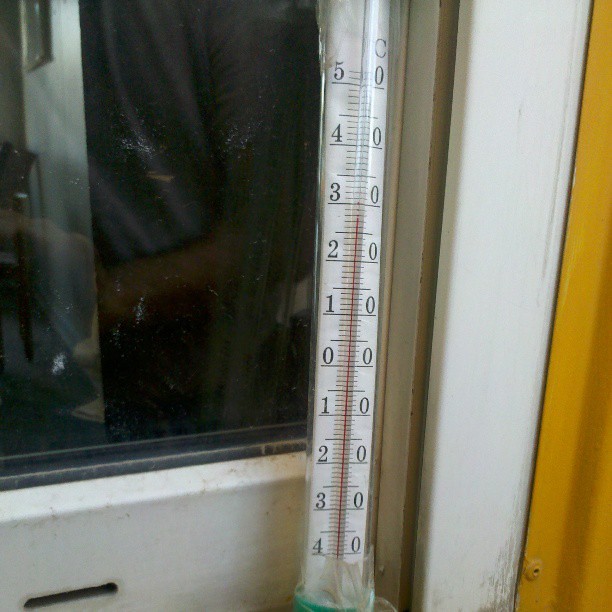This is a color indoor photograph with an almost perfect square aspect ratio, capturing a zoomed-in section of a room, particularly a corner beside a window. 

The lower left half of the image displays a white window sill and the solid framing of the window. Above this, occupying about half of the picture and extending to the top, is a dark, shiny surface, likely part of the window or a piece of metal that reflects some light.

Centrally positioned, a large thermometer descends from the middle top to the middle bottom of the image. The thermometer is white with black markings, calibrated in Celsius. Its scale starts at 50 degrees, decreasing to 0 degrees and further down to -40 degrees. The temperature reading indicated by a red line shows approximately 30 degrees Celsius. At the bottom end, the thermometer is partially wrapped with something, revealing a hint of green at the base before disappearing out of the frame.

Adjacent to the thermometer, a small wooden panel is visible, leading up to a white-painted wooden board. To the side, a sliver of a natural wood-colored door is faintly noticeable, contributing to the intricate details in this close-up, indoor capture.